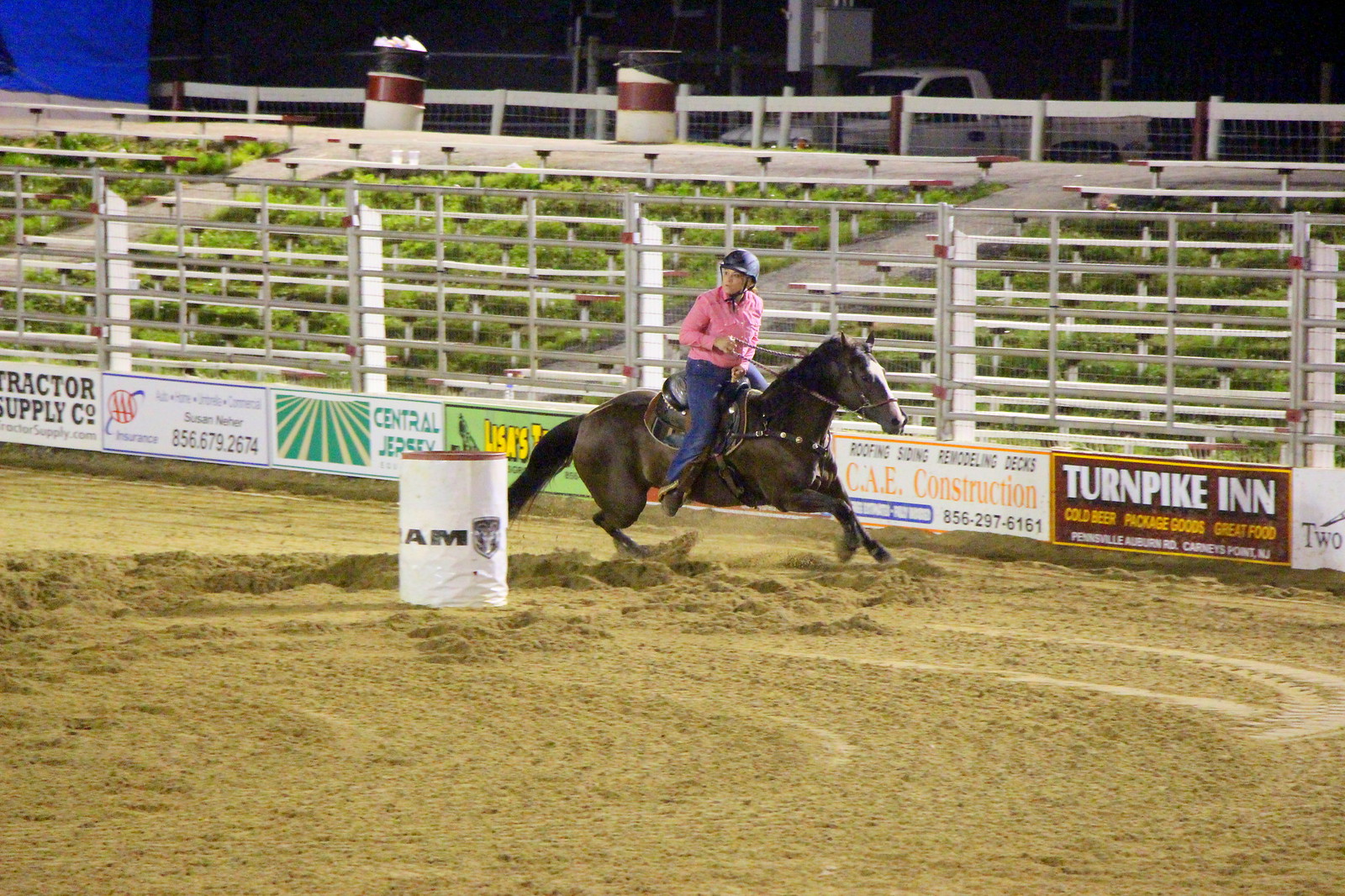This photograph captures an outdoor nighttime rodeo scene, featuring a woman in the center riding a dark brown horse with a distinctive white stripe down its face. The rider, wearing a black helmet, pink long-sleeve shirt, and blue jeans, guides the horse around a white barrel marked with the letters 'AM' and what appears to be a Dodge logo. The action takes place on a dirt or sandy surface, possibly a horse track or corral within a stadium setting. Surrounding the arena, a metal fence adorned with various advertisements from sponsors like Tractor Supply Company and Turnpike Inn is visible. Beyond the fencing, there are empty spectator benches on grassy ground, indicating the area is currently unoccupied, perhaps due to it being a practice session. Further back, a white truck is parked, and the sky above is dark, further emphasizing the late hour of the event.